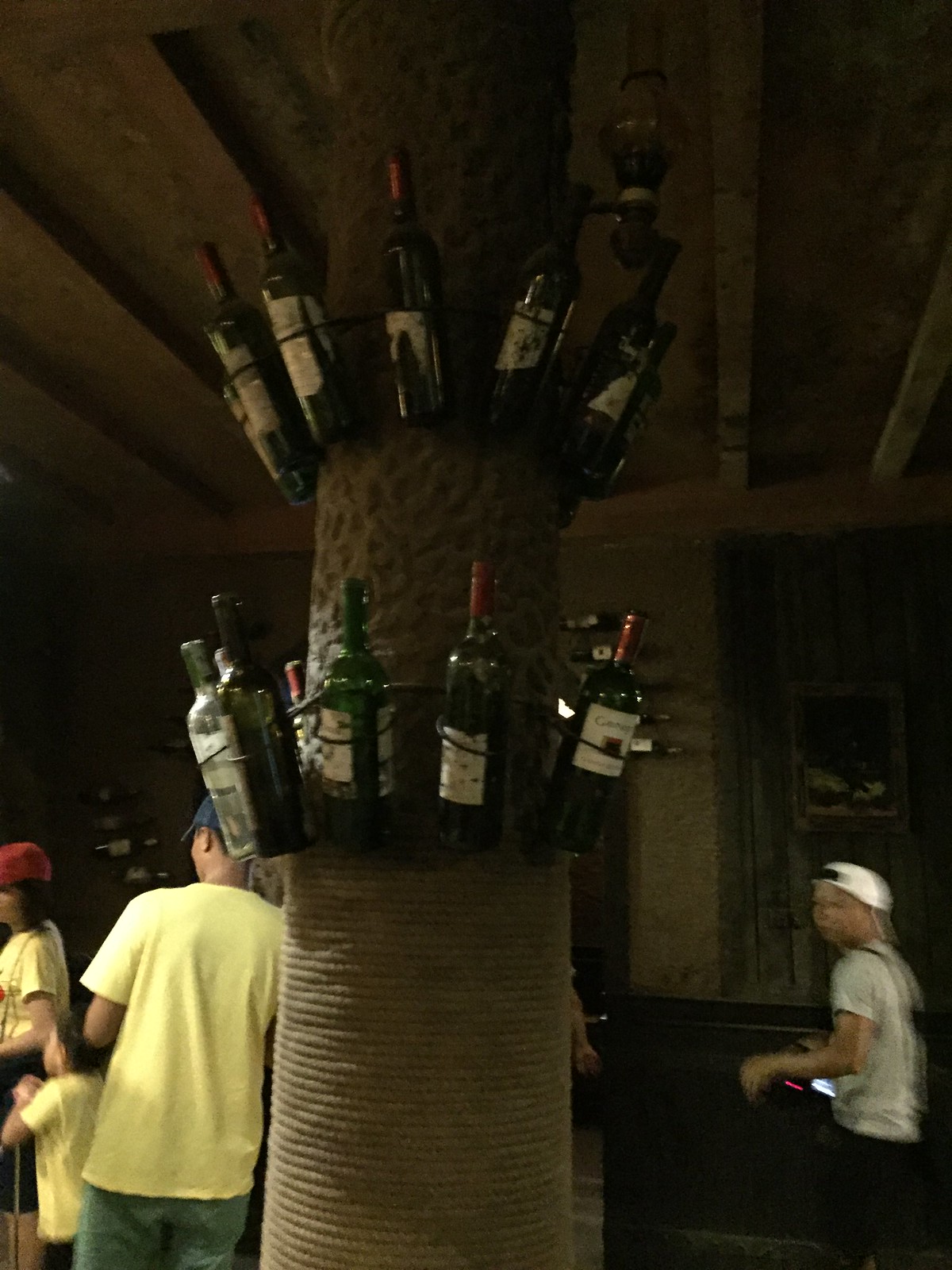The photo showcases the interior of a building dominated by a large, brown pillar that extends from the floor to the dark wood-beamed ceiling. The pillar is adorned with two circular racks of wine bottles, one positioned high and the other low. The green bottles feature white labels and shiny red metal stickers around the tops where the lids are. To the left, a person in a blue hat, t-shirt, and jeans stands next to a child in a similarly colored shirt. Further left, another child wears a matching t-shirt with basketball shorts and a red hat. On the right, another child in a white baseball hat and gray t-shirt holds a phone. The back wall and the right side of the photo are lined with more wine bottles. The scene includes one adult and several children, all congregated around an array of alcoholic beverages, which adds a curious and slightly unsettling dynamic.